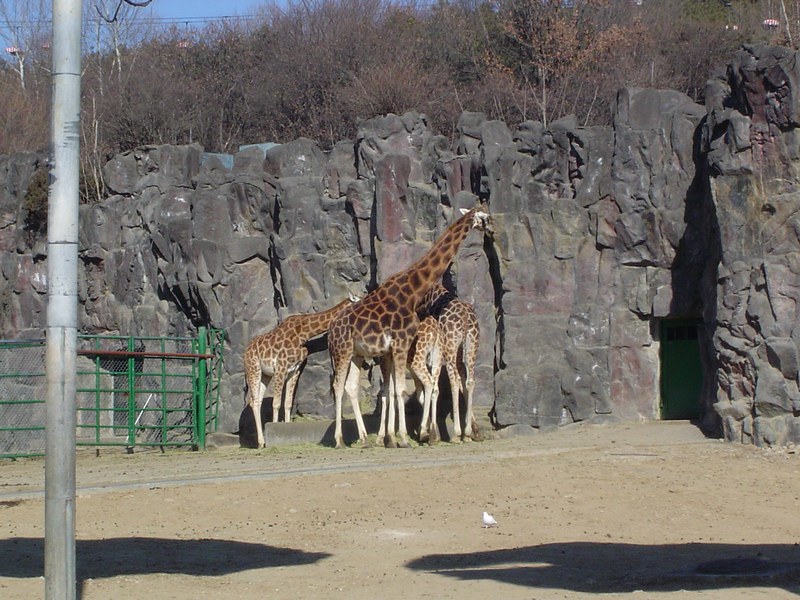This image captures a zoo habitat for giraffes, featuring four giraffes in the center. One giraffe stands on a rock, facing right, showcasing its brown fur with dark spots and white underside and legs. Two more giraffes are partially visible in the background, showing mostly their backs, while the fourth giraffe stands near them. The setting includes tall, rocky, black, burgundy, and tan walls at the back, with dry shrubbery above. In the foreground, the ground is a light tan dirt. On the left side, there is a green metal gate with wheels and a pole that presumably holds an umbrella, casting a shadow. Additionally, a green iron railing is visible to the mid-left. In the distance, a skyline or aerial tramway suggests a means to traverse the park. Shadows of giraffes stretch across the ground in the foreground, adding depth to the scene.